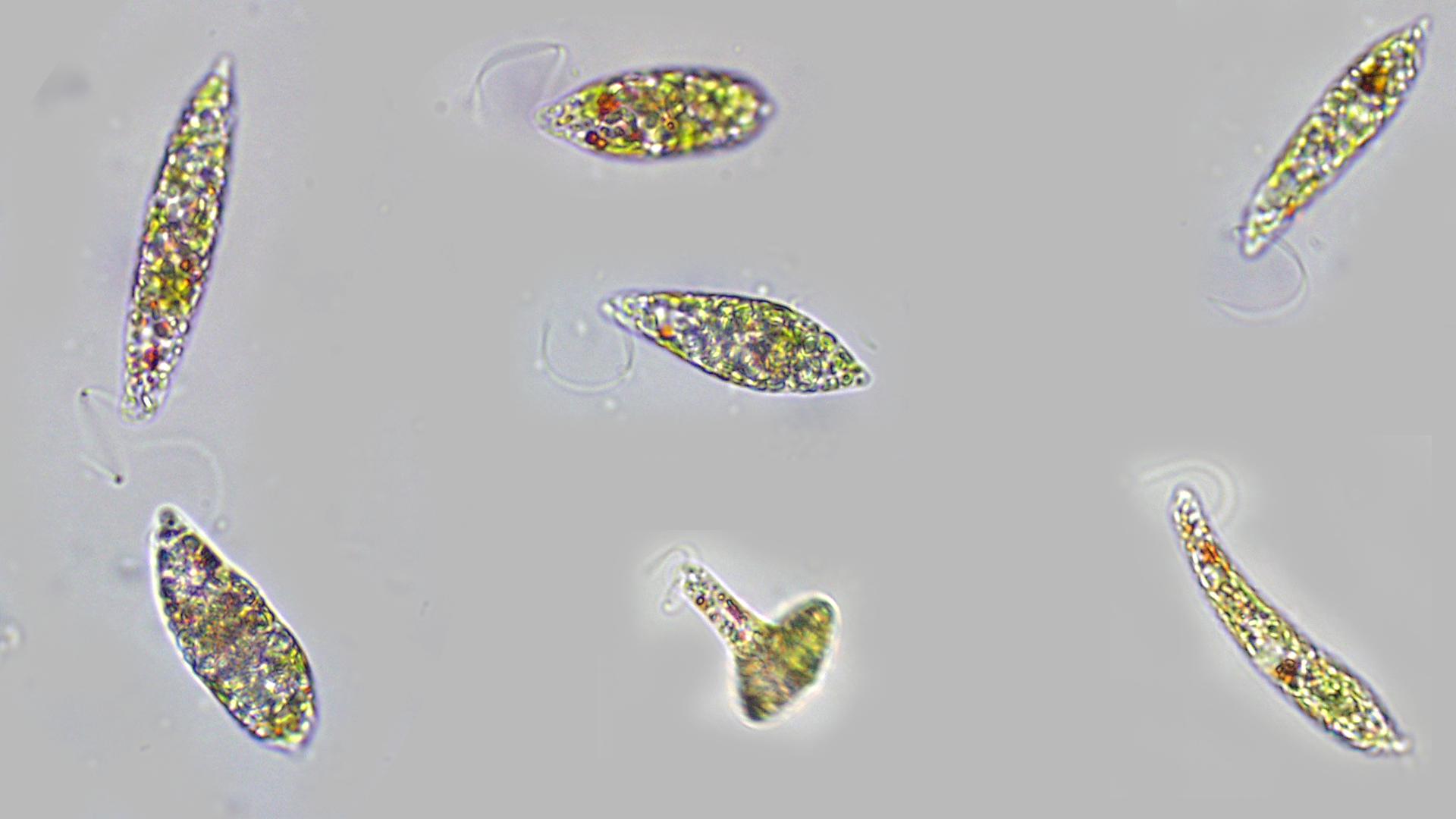This image depicts a microscopic view of several diverse cells, each with unique shapes and vibrant internal colors, resembling stained glass art set against a gray background. There are seven primary cells in the frame:

- On the right side, two cells are elongated and thin, reminiscent of germ-like structures, featuring a combination of glittery greens, blues, and reds within their mostly clear bodies. 
- In the center, three cells stand out: one with an odd, almost irregular shape, another roundish, and the last one shaped remarkably like a beaker with a wide base narrowing to a spout at the top. The internal colors vary, with a visually striking mix of yellow, red, blue, and white.
- On the left side, two more elongated cells are noticed, one resembling a long bean with swirling colors of yellow and red inside, and another cell with blue, yellow, and red hues, designed similarly to a boat.

The entire scene is set against a gray backdrop, enhancing the colorful, shimmering internal structures of these uniquely shaped cells.